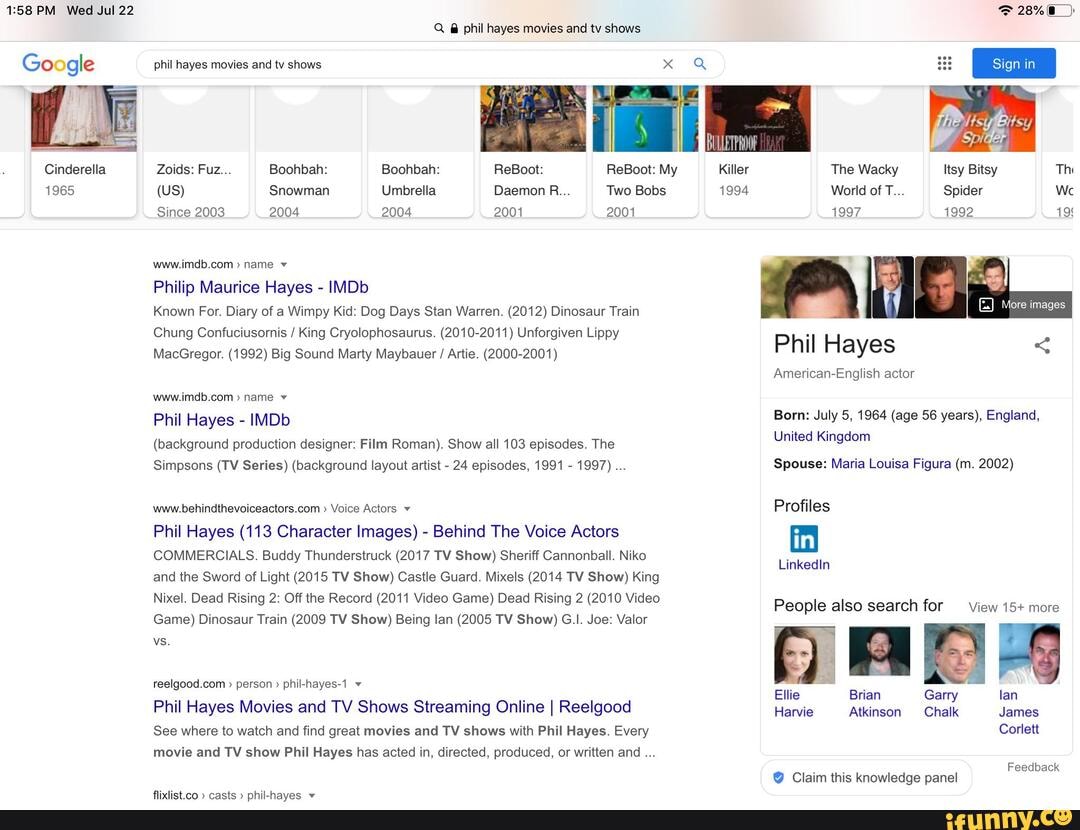The image depicts a Google search results page for "Phil Hayes movies and TV shows." At the top of the page, there is a horizontal banner displaying various movies and TV shows featuring Phil Hayes, organized chronologically from his earliest to most recent works, left to right. On the right side of the page, there is a section providing general information about Phil Hayes, including details such as his birth date, place of birth, spouse, and a link to his LinkedIn profile. The main section of the page shows four search results focused on Phil Hayes, with the first two results sourced from IMDb, the widely known movie and television database.